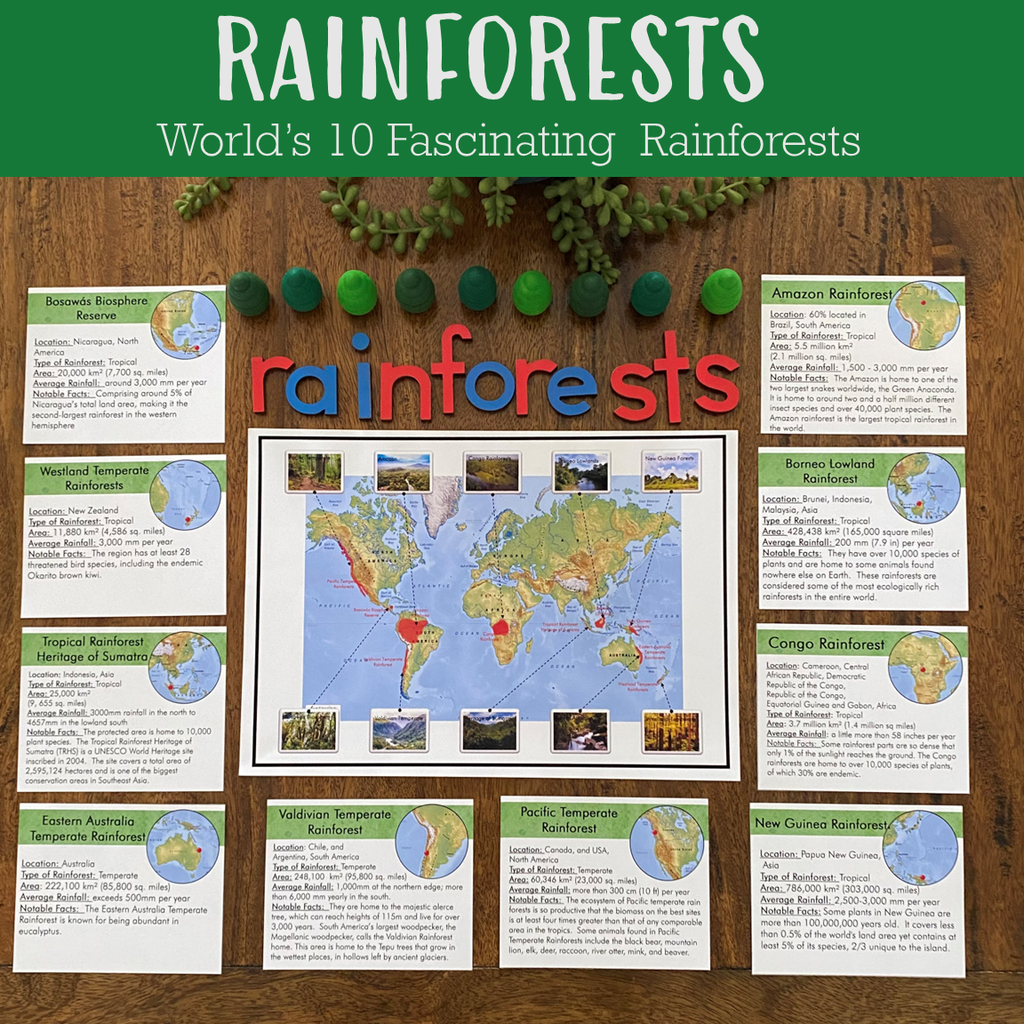The photograph showcases a detailed educational display about rainforests mounted on a brown wooden wall covered with panels. At the top, bold and colorful letters alternate in red and blue to spell out "Rainforests," accompanied by the subtitle "World's 10 Fascinating Rainforests." Centrally featured is a large world map, around which are arranged ten index card-like pieces of information, each representing a different rainforest. Notable spots include the Bazaawa Spire Sphere Reserve in Nicaragua and the Westland Temperate Rainforests in New Zealand. Each card provides extensive details such as location, type, area, average rainfall, and notable facts about the rainforests, including biodiversity statistics like threatened species. The various cards are pinned to the wooden backboard, and smaller pins represent the specific locations on the globe. Despite the small and somewhat hard-to-read font, the overall image is vivid and clear, effectively conveying an in-depth overview of some of the world's most significant rainforests.